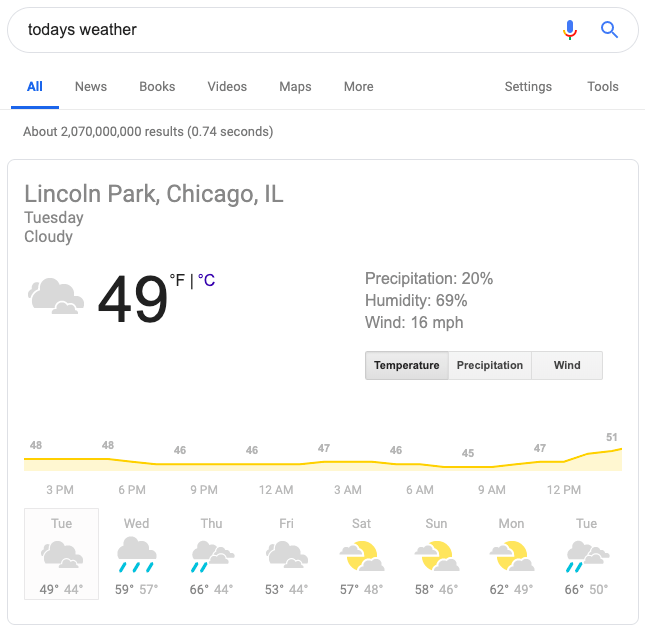Here is a cleaned-up and detailed caption for the image:

---

**Detailed Weather Forecast Screenshot for Lincoln Park, Chicago, IL**

This screenshot captures the results of a Google search for today's weather in Lincoln Park, a neighborhood in Chicago, Illinois. The search yielded approximately 2,070,000 results in 0.74 seconds. The display is slightly cropped and showcases weather conditions specifically for Tuesday.

The primary information indicates that the weather is currently cloudy, with a corresponding image of gray clouds. The temperature is shown as 49 degrees Fahrenheit, with an option to convert it to Celsius via a clickable blue "C." Additional weather metrics include a 20% chance of precipitation, 69% humidity, and winds blowing at 16 miles per hour.

Further down, there's an option to view data on temperature, precipitation, or wind. Currently, the temperature data is selected, displaying an hourly forecast spanning from 3 p.m. to 12 p.m. the following day. Temperatures range from a high of 48 degrees at 3 p.m. to a low of 45 degrees at 6 a.m., eventually rising to 51 degrees by noon on Wednesday.

Following this hourly breakdown, a more extended forecast for the week is provided:

- **Wednesday:** Rainy, with temperatures reaching a high of 59 degrees and a low of 57 degrees.
- **Thursday:** Rainy again, with a high of 66 degrees and a low of 44 degrees.
- **Friday:** Cloudy, with a high of 53 degrees and a low of 44 degrees.
- **Saturday:** Partly cloudy with sunny intervals, high of 57 degrees, and a low of 48 degrees.
- **Sunday:** Partly cloudy with sunny intervals, high of 58 degrees, and a low of 46 degrees.
- **Monday:** Partly cloudy with sunny intervals, high of 62 degrees, and a low of 49 degrees.
- **Tuesday:** Overcast with rain, high of 66 degrees, and a low of 50 degrees.

Overall, this screenshot provides a comprehensive look at the weather forecast for the upcoming week in Lincoln Park, illustrating a variety of conditions ranging from cloudy and rainy to partly sunny days.